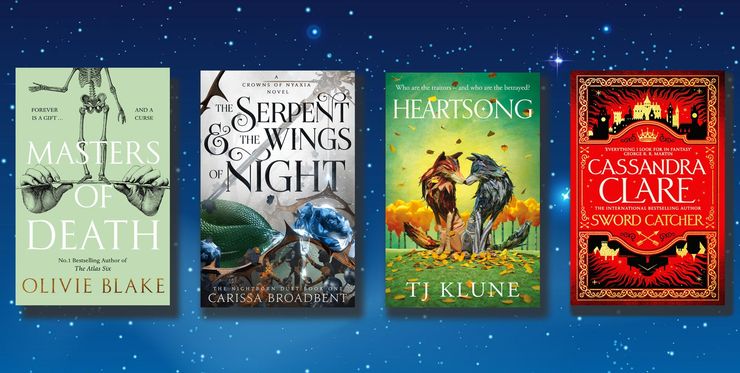The image features four distinct books arranged side by side against a night sky background adorned with stars. The upper part of the backdrop is a dark midnight blue, gradually transitioning to a lighter blue towards the bottom, with stars of various sizes and brightness scattered across.

From left to right, the first book is "Masters of Death" by Olivia Blake. Its cover is a muted mint color, depicting a skeleton from the shoulders down, holding an object resembling a pencil or thin rod.

The second book, "The Serpent and the Wings of Night" by Carissa Broadbent, has a cover with a serpent and dark, thorny elements, featuring shades of green and blue.

Next is "Heart Song" by T.J. Klune, a green book with illustrations of two wolves facing each other against a backdrop of yellow-tinted trees and grass. One wolf is brown with a white muzzle, while the other is black with gray legs and a gray muzzle.

The final book, "Sword Catcher" by Cassandra Clare, has a red cover featuring a small castle-like structure surrounded by what appears to be flames.